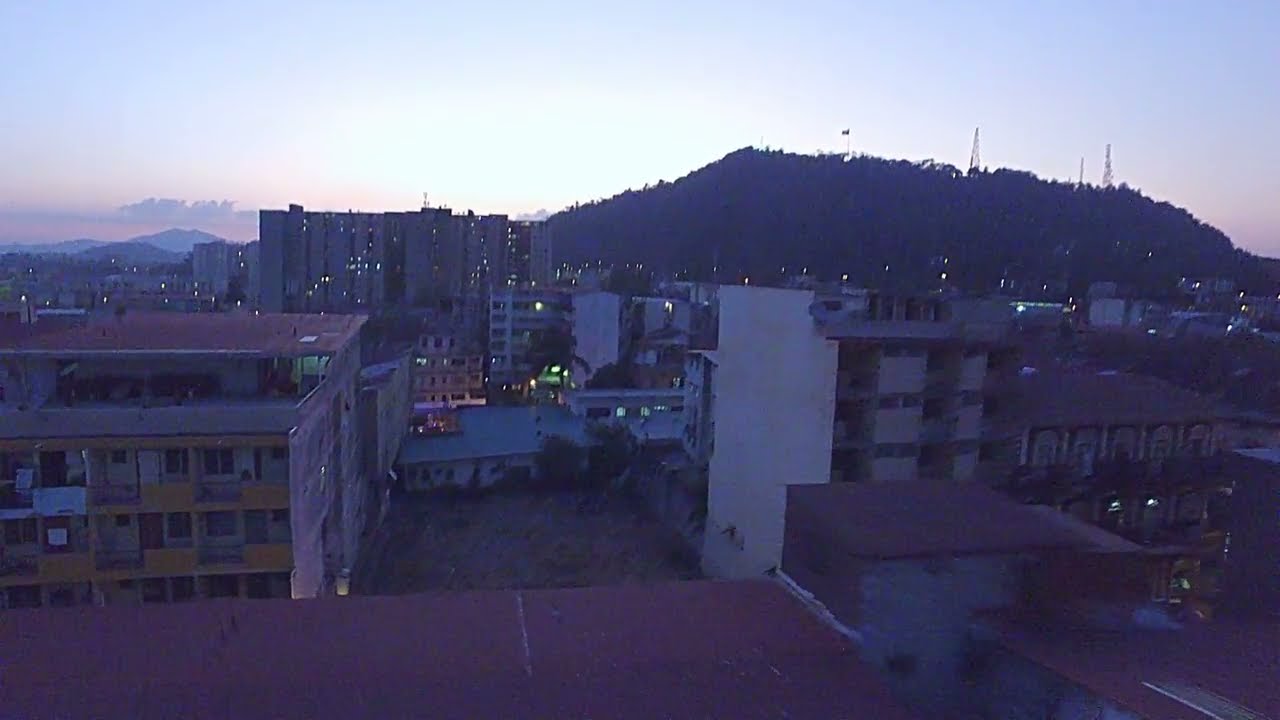The image depicts a cityscape characterized by a mix of dilapidated buildings and distant, modern structures under a hazy twilight sky. In the foreground on the left, there is a large, rundown building with a red roof extending across a significant portion of the image, showcasing balconies and multiple stories that look weathered and unkempt. Further behind, there is a noticeable gap leading to another similarly dilapidated structure. Towards the horizon, larger and relatively newer buildings rise, their windows illuminated, adding contrast against the older facades in the immediate view. A hillside can be seen in the distance, crowned with trees and possibly a flag, standing against a backdrop of dark mountains. The sky appears grayish, with hints of orange near the horizon, indicating the setting sun and bathing the scene in a twilight glow. Scattered lights and indistinct buildings blend into the scenery, completed by a suggestion of construction cranes hinting at ongoing development.